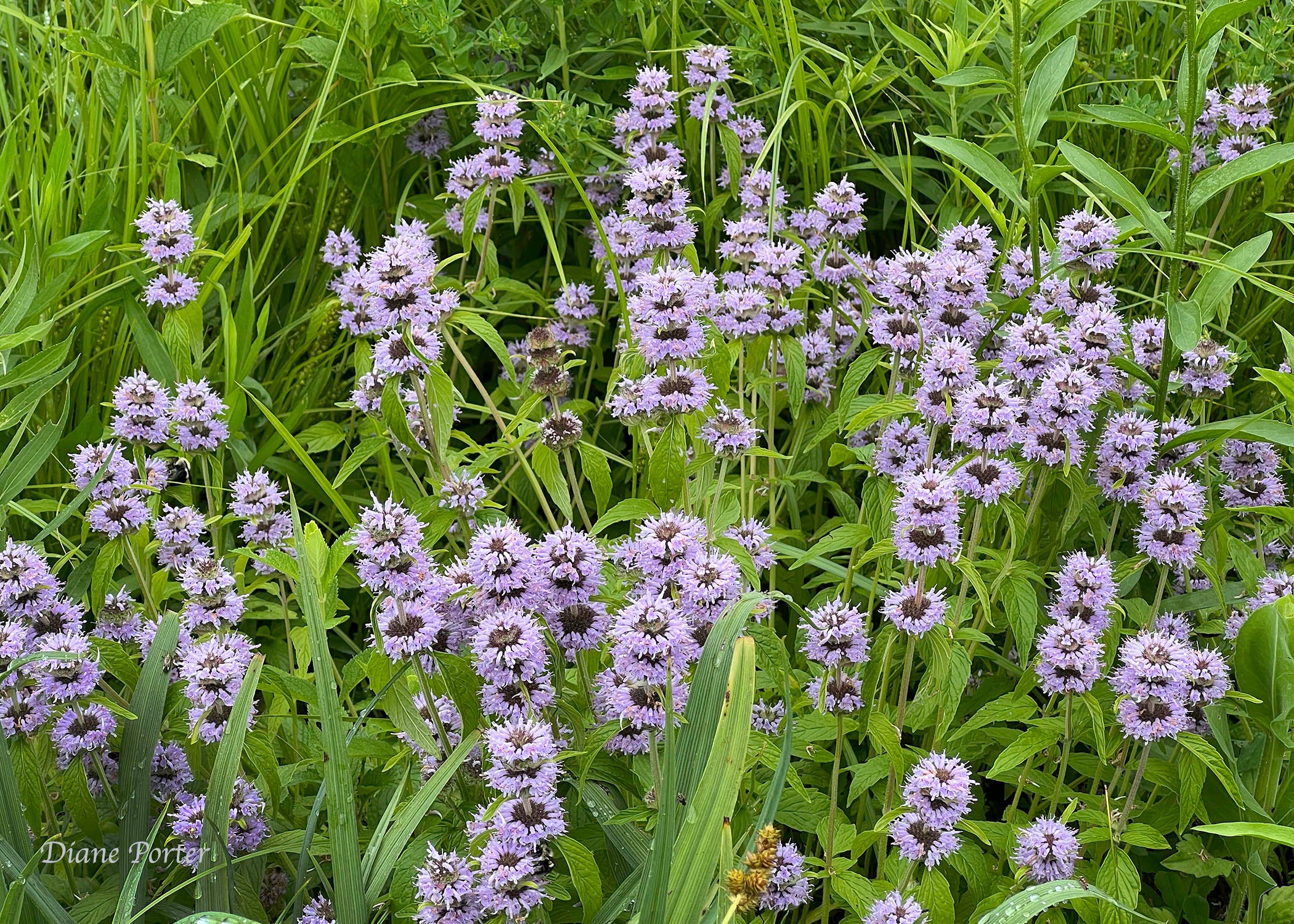This professional photograph by Diane Porter, as indicated by the white text in the lower left-hand corner, captures a lush, green field adorned with numerous light purple flowers. The flowers, resembling daisies, are bunched in clusters along singular stems, with some displaying a darker purple center. Amidst the sea of purple blossoms, green grasses and leaves fill the scene, contributing to the vibrant, springtime ambiance. The wildflowers and varied grass lengths create a meadow-like setting, emphasizing the natural beauty of the landscape.